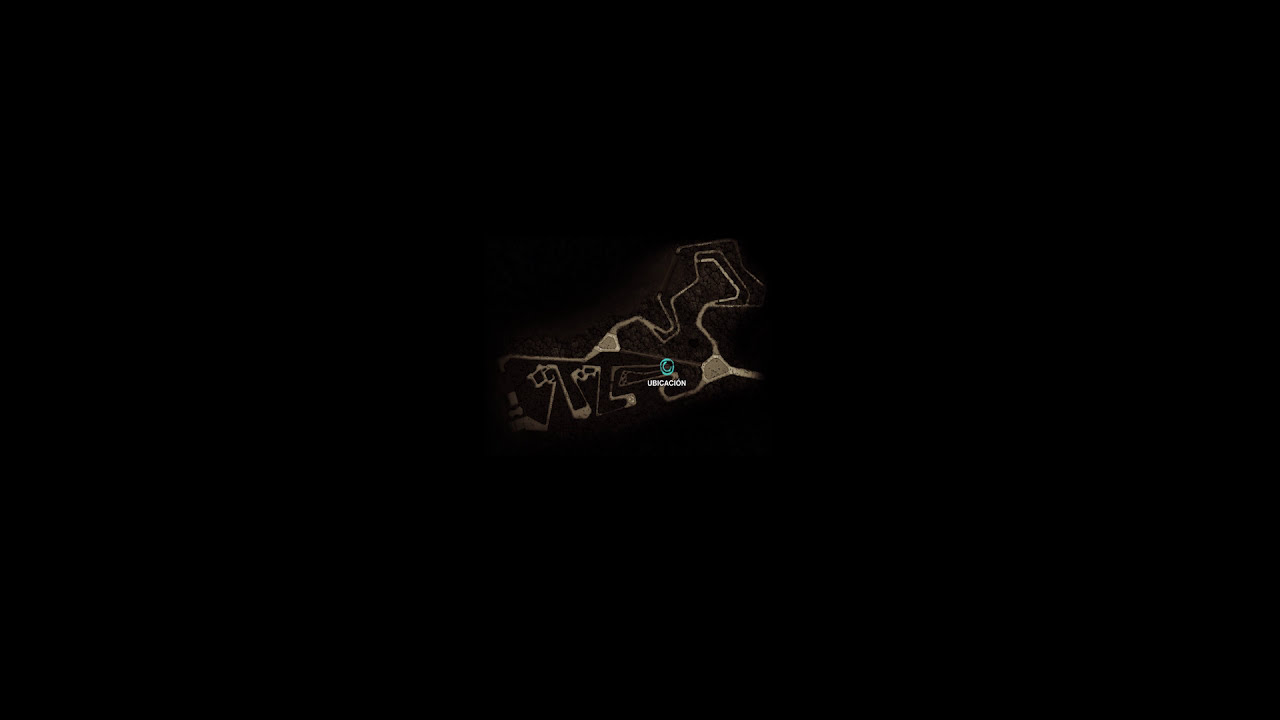The image is a horizontal 16 by 9 composition dominated by a pitch-black background. At the very center, an abstract, graffiti-like series of tan and gold-gray lines glistens brightly against the darkness, suggesting an artistically drawn map or road network. Nestled at the heart of this intricate design is a small turquoise-green circle, which could be interpreted as a company watermark. Beneath this circle, in crisp white uppercase letters, reads "UBICACION." The design, reminiscent of illuminated drawings on a Light Brite, occupies only about 10% of the entire black canvas, leaving the rest enveloped in deep, uninterrupted blackness.